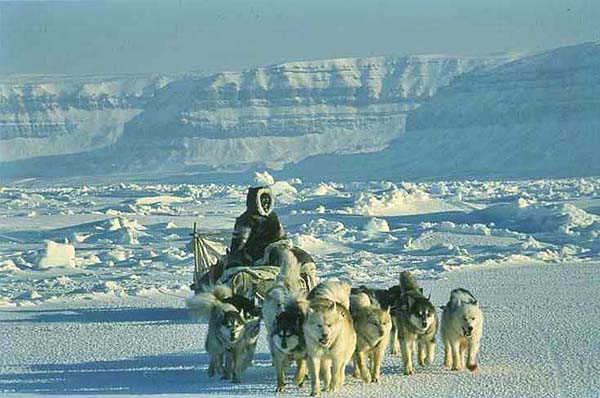In this captivating image, an expansive, snow-covered wilderness stretches under a clear blue sky, reminiscent of the Arctic or Alaskan terrain. Majestic mountain ranges, blanketed in pristine white snow, dominate the background, devoid of any visible vegetation or structures. In the middle of the scene, a man, bundled up in a heavy fur-lined Eskimo parka, stands on a sled. His face is obscured by the hood, emphasizing the harsh, frigid conditions. Leading the charge are seven, possibly eight, sturdy huskies. These sled dogs, with their diverse fur colors ranging from white to dark shades of gray and black, are harnessed in front of the sled, ready to navigate the icy expanse. The entire ensemble captures a moment of resilience and adventure in one of nature's most formidable environments.